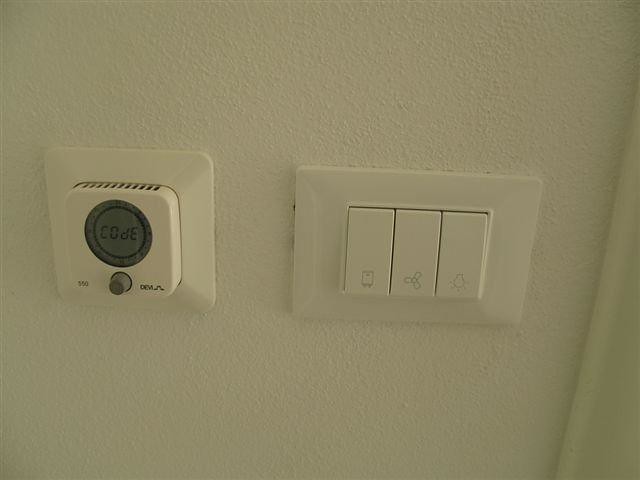The image features a white stucco wall with a notably textured, bumpy surface. Dominating the center of the image are two distinct sets of control panels.

On the far left, the first panel is square-shaped with a protruding cube. The top of this cube has ventilation holes, and towards the bottom, it bears the number "360" or "350." A gray, knob-like button, reminiscent of a radio volume control, is also present and marked with the word "DEVLA." Above this, there is a gray circular ring and a digital display that reads "CODE," suggesting a possible error or alert.

The second panel is rectangular and situated to the right of the first. It features three horizontal buttons centrally located within the rectangle. The buttons are illustrated with icons: the first appears to be a clipboard or manual, the second depicts a three-bladed ceiling fan, and the third shows a light bulb with rays indicating it is turned on. It's inferred that these buttons could potentially control power, a ceiling fan, and a light respectively.

Overall, the image portrays part of two control panels likely responsible for managing an air conditioner, lighting, and a ceiling fan within the household.